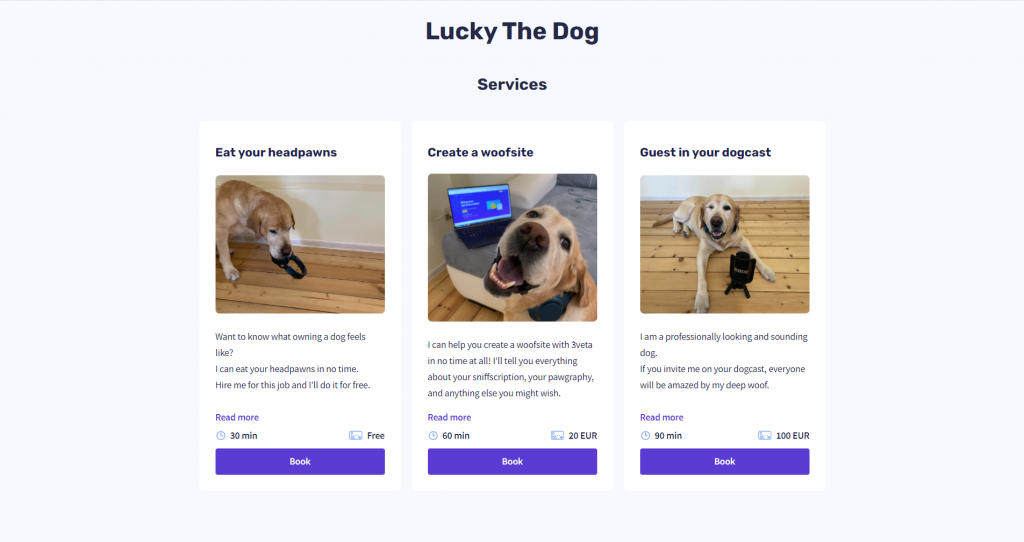**Detailed Description:**

The image features a promotional poster for a service-providing dog named Lucky. At the very top center of the poster, the text reads "Lucky the Dog" in black font. Below that, the services offered by Lucky are presented within three white boxes on a grayish-white background.

1. **Service 1: Eat Your Headphones**
   - **Visual:** A picture of Lucky chewing on a pair of headphones.
   - **Description:** "Want to know what owning a dog feels like? I can eat your headphones in no time. Hire me for this job and I'll do it for free."
   - **Additional Info:** Below the description is a link option in periwinkle-colored font that says "Read More." There's an icon of a clock indicating a 30-minute duration. The service is free of charge. A periwinkle-colored box with white font reads "Book."

2. **Service 2: Create a Website**
   - **Visual:** Lucky the Dog is seen with a laptop, looking into the camera and smiling.
   - **Description:** "I can help you create a website with three vita in no time at all. I'll tell you everything about your sniffscription, your pawgraphy, and anything else you might wish."
   - **Additional Info:** A "Read More" option is available. The service duration is 60 minutes, and it costs 20 euros. The "Book" button is likewise present.

3. **Service 3: Guest in Your Dogcast**
   - **Visual:** Lucky with a microphone, ready to speak in a podcast.
   - **Description:** "I am a professionally looking and sounding dog. If you invite me on your dogcast, everyone will be amazed by my deep wolf."
   - **Additional Info:** A "Read More" button is included. The session lasts 90 minutes and costs 100 euros. The "Book" button is available for scheduling.

Each service box is designed uniformly with a "Book" button in a periwinkle-colored box with white font, facilitating easy action to engage Lucky’s services.